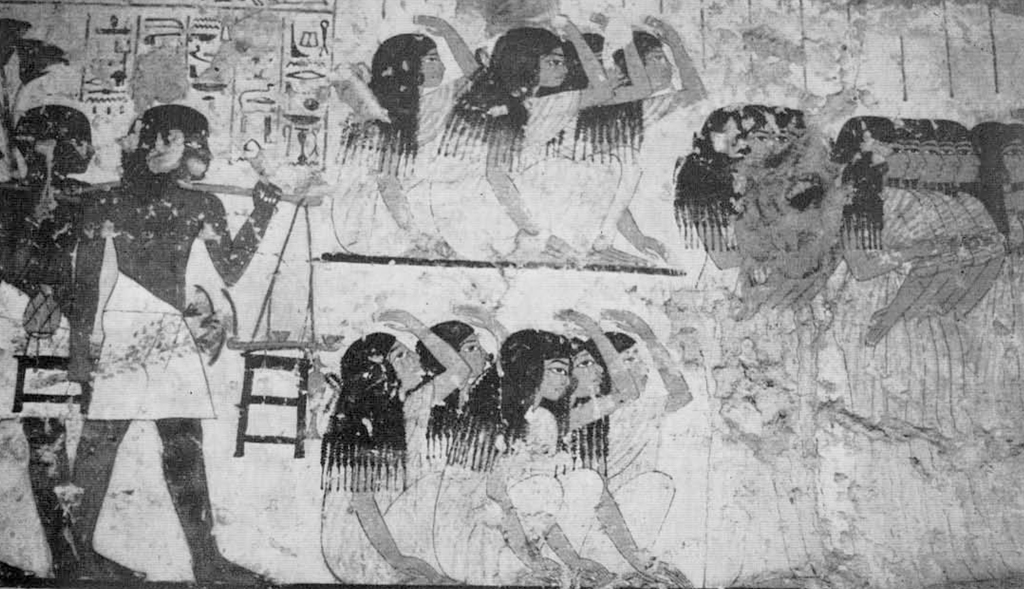This black-and-white photograph showcases an ancient Egyptian scene. The weathered surface features detailed hieroglyphics to one side, indicating its historical significance. Central to the composition are Egyptian men, garbed in toga-like white outfits, carrying a long wooden pole with a stool-like object hanging from it. Surrounding them, several Egyptian women with long, dark hair are kneeling, also dressed in white. Some of the women have their arms partially over their heads, perhaps gesturing or in prayer. The image shows signs of aging and deterioration, with noticeable chipping and missing chunks, which adds a haunting sense of antiquity to the artwork.